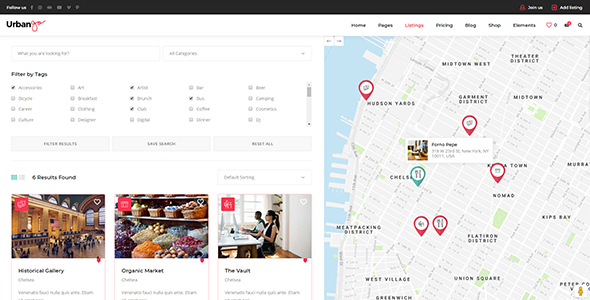The image features a detailed layout with various elements and text arranged in a structured manner. At the top, there is a small black rectangle with white text on the left-hand side. Adjacent to it, on the right-hand side, there are two red symbols, each accompanied by white text.

Beneath this, the word "Urban" appears in black, followed by an indeterminate red word. On the right, a block of text is predominantly in black, except for the third word from the left, which is in red. Accompanying this text are several symbols, including a heart, a dot, an indistinguishable symbol, and possibly a magnifying glass.

To the left below this section, there is a gray line leading to two gray outlined rectangles containing text. Underneath these rectangles is additional text, possibly with check marks or boxes for check marks, though it is difficult to discern due to the small size.

Following this are three gray rectangles with writing within them. Adjacent to these, there is a small blue square and a small gray square, each containing text. Below these squares, there are three images with captions beneath each one, although the exact content of the images is unclear.

On the right-hand side of the image, there is a map featuring several symbols in red and one in green. Embedded within the map is a white rectangle containing a picture and text to the right of the picture.